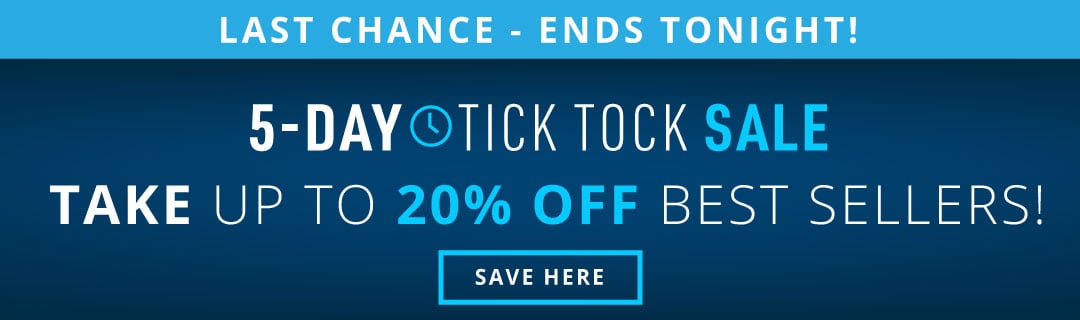This is a detailed description of a portion of a print advertisement with a vibrant and eye-catching design. 

At the very top, there is a thin, electric blue horizontal box. Inside, in all-capital white letters, it reads: "LAST CHANCE - ENDS TONIGHT!"

Beneath this, there is a larger navy blue box. In bold white font, it states: "5-DAY," followed by an electric blue clock icon. Next to the icon, in all-capital letters, it says: "SALE." The combination of bold and non-bold text in varying colors emphasizes the urgency and excitement.

The next line continues the variation in font styles and colors. It reads: "Take up to 20% off bestsellers!" Here, "Take" is in bold white font, "up to" is in non-bold white font, "20% off" is in bold electric blue font, and "bestsellers!" is in non-bold white font. 

At the bottom, there is an electric blue box outline with a navy blue fill, matching the background. Inside this outlined box, in white type font, it reads: "SAVE HERE." This text indicates a clickable button designed to direct the reader to the sale.

The overall design effectively uses color contrast and varied typography to draw attention and create a sense of urgency for the sale events.